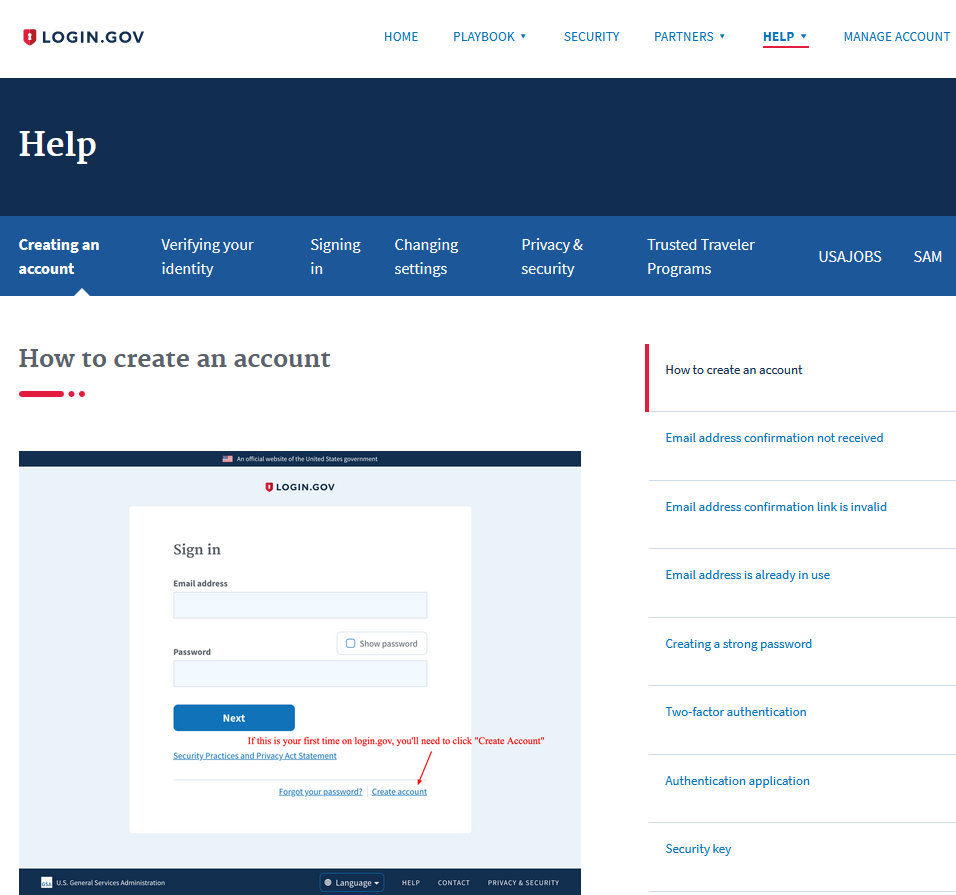This is a screenshot of a website's help section. The background at the top is predominantly white, featuring a white bar in the upper left corner. Adjacent to this bar is a prominent red shield icon with the number "1" inside it, placed next to bold black text that reads "login.gov." 

To the right of this section, there are a series of clickable links in blue font: Home, Playbook (which is a drop-down menu), Security, Partners (also a drop-down menu), Help (another drop-down menu), and Manage Account. The "Help" link has been selected in this instance. 

Beneath this navigation bar, a dark blue rectangle spans the width of the screen, displaying the word "Help" in white text. Directly below, there's a lighter blue rectangle containing several white-font options. The options listed include "Creating an account" (which is currently selected), "Verifying your identity," "Signing in," "Changing settings," "Privacy and security," "Trusted traveler programs," "USA jobs," and "SAM."

Further down, the main content area of the page is white. On the right side, there appears to be a vertical menu that allows selection of different pages to view on the left. At the top of this vertical menu, the option "How to create an account" is selected and displayed in black font. Below this, additional categories or help topics are listed in blue font: "Email address confirmation not received," "Email address confirmation link is invalid," and "Email address is already in use."